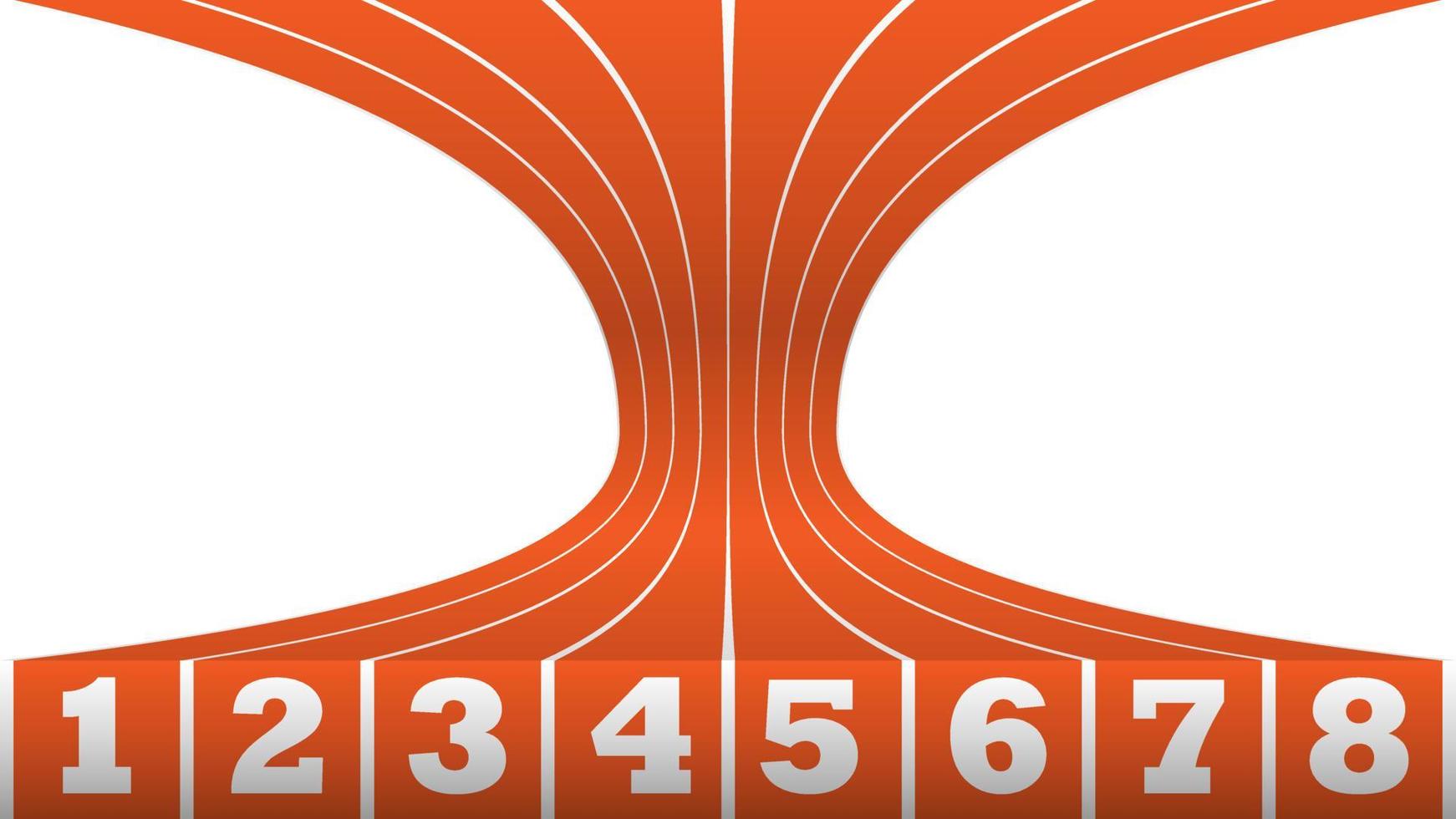The image features a vibrant and clear graphic set against a solid white background, showcasing the numbers 1 through 8 positioned along the bottom. The focal point of the graphic is a red-orange swirling, hourglass-shaped pattern characterized by its thin middle section which expands outward into a more pronounced, wide form at both ends. This pattern is flanked by thin curved lines that guide the eye along its shape, converging towards the center before curving upwards. Thin white vertical lines act as dividers between the numbers at the bottom, creating a balanced visual structure. The red-orange lanes create an optical illusion, making the top lines appear thinner than the bottom ones. Additionally, white half-oval shapes are positioned on the left and right of the central swirl, contributing to the intricate design. The overall illustration is brightly lit, making all details sharply discernible.